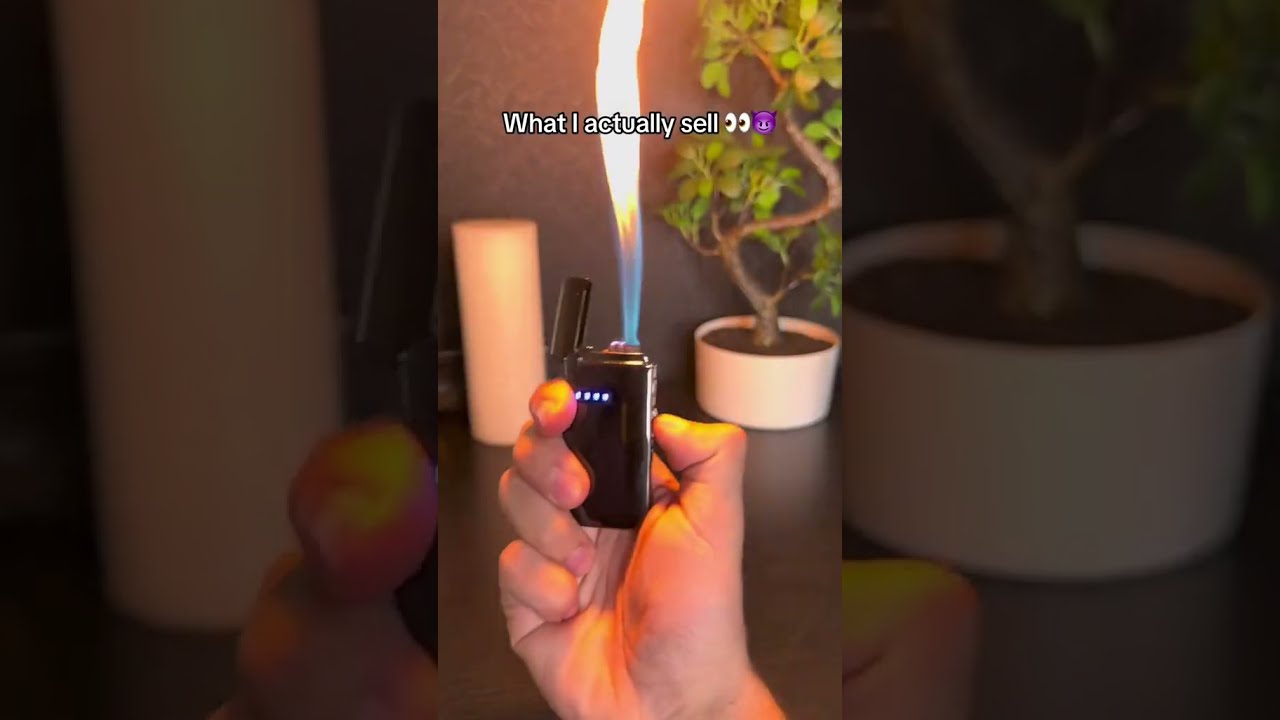In the image, a person's right hand is prominently featured at the bottom center, firmly gripping a black, rectangular butane lighter. The lighter is ignited, producing an impressive flame that transitions from a bright blue at the base to a vivid yellow and white at the top. Above the image, the text reads "What I actually sell," accompanied by eye emojis and a purple devil emoji. 

The background showcases a slightly blurry, faded scene on a grayish wall, which includes a brown surface holding a white cylindrical planter. Inside the planter, there's a small bonsai tree with a curvy trunk and vibrant green leaves. Adjacent to it is an unlit candle. The entire scene is horizontally aligned, with the lighter's flame standing out as the focal point against the subdued backdrop.